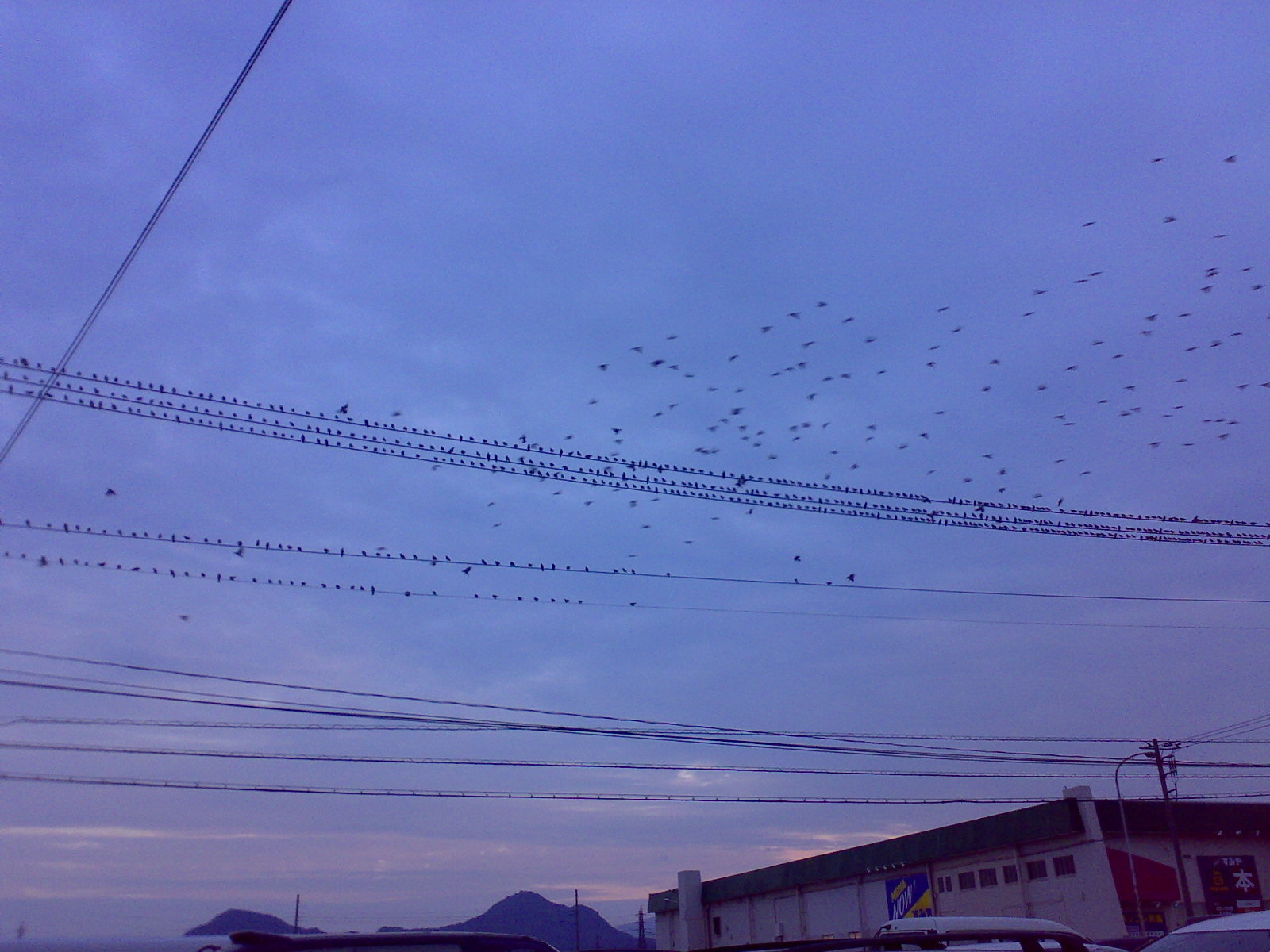An outdoor photograph captures a dusky sky transitioning from blue to purplish with hints of pink, slightly dimming as evening approaches. The backdrop is densely covered with thin clouds, lending a textured canvas overhead. Several power lines stretch horizontally across the image, some intersecting mid-way with vertical or diagonal lines. These lines host a large flock of small black birds, with many perched densely together and others fluttering into the sky. In the bottom section of the image, rolling hills recede into the distance, and a white building with a black roof is visible in the bottom right corner. The building features some red designs and is partially obstructed by a blue and yellow sign and the rooftops of a few vehicles. The full picture conveys a peaceful, almost surreal twilight moment blending natural and man-made elements.